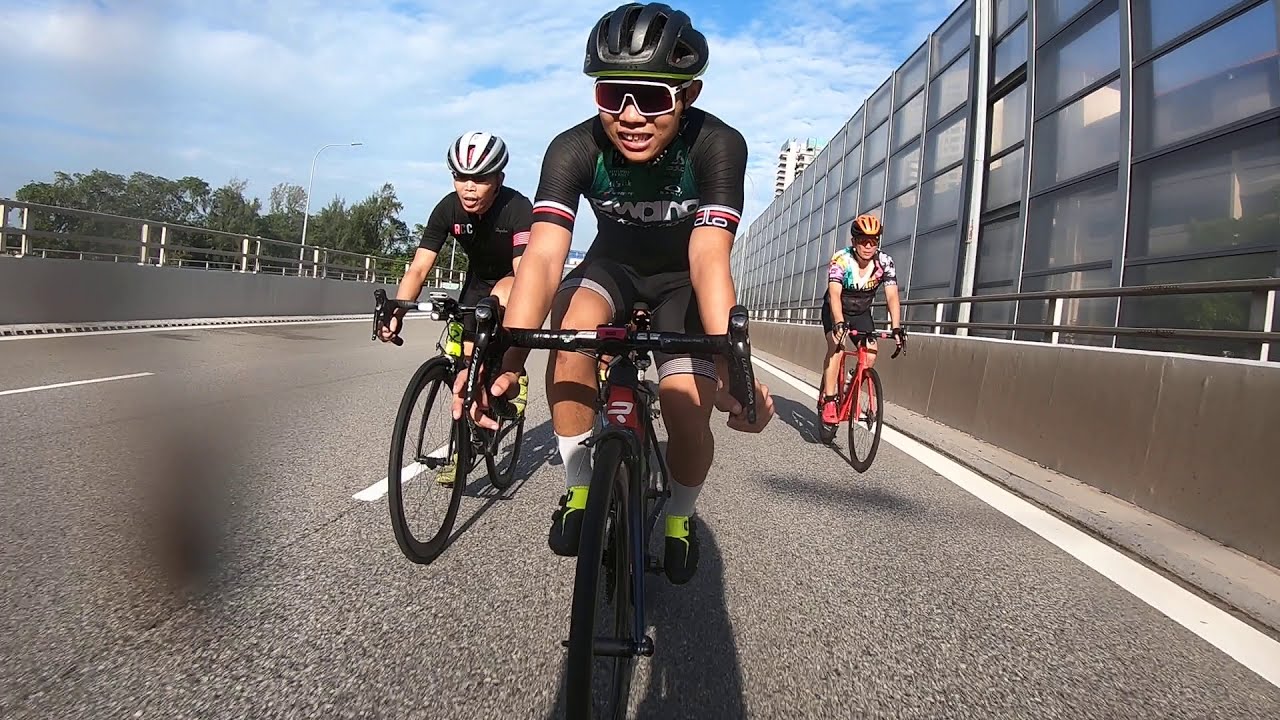This photograph captures three Asian men intensely racing on a three-lane highway. Each biker is clad in race-specific gear including helmets, sunglasses, and tight-fitting jerseys. The central figure, closest to the camera, sports a black racing outfit, a black helmet, and white sunglasses, with high white socks and black shoes. Flanking him on the left, the second biker wears a black ensemble similar to the central racer, with a white helmet. The third racer, positioned further back on the right, stands out in a mixed outfit featuring black shorts and a distinctive white top with yellow and orange accents, along with an orange cap. Both the left and right bikers have either red or black bikes and are hunched forward over their curved handlebars, indicative of a competitive pace.

The setting is a paved road bordered by metal guardrails and concrete barriers, each topped with metal railings. To the right, there is a striking building with an extensive facade of glass windows, while the left side of the image contains what appears to be a smear or a dark, obscure mark. The photograph appears to be taken from a following vehicle—possibly another bike or a car—capturing the dynamic motion of the race.